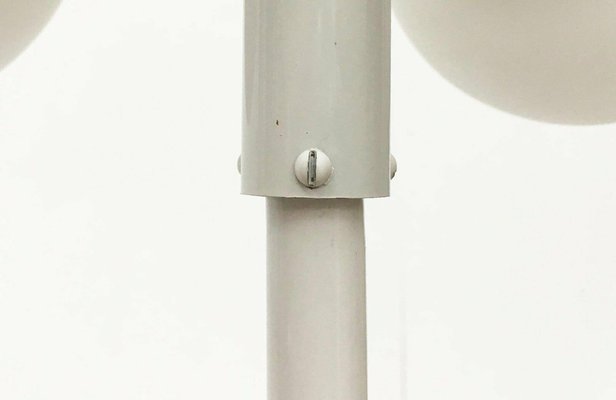The image features a close-up of a metal structure consisting of two cylindrical tubes, with a narrower lower pole slotted into a thicker upper pole. The entire scene is bathed in a light gray color. The larger, top tube has three screws visible: one centrally placed flat head screw, painted off-white like the tubes and distinctly darker at its vertical slot, and two additional screws positioned on the left and right. The background is an off-white, with an unidentifiable gray section in the top and left corners. Two semi-visible circular objects of the same color as the tubes appear at the top left and top right, respectively, adding to the mystique of the photograph. Though the exact function of the metal structure remains unclear due to the close-up nature of the shot, it gives the impression of being a leg or a supportive bar of furniture.